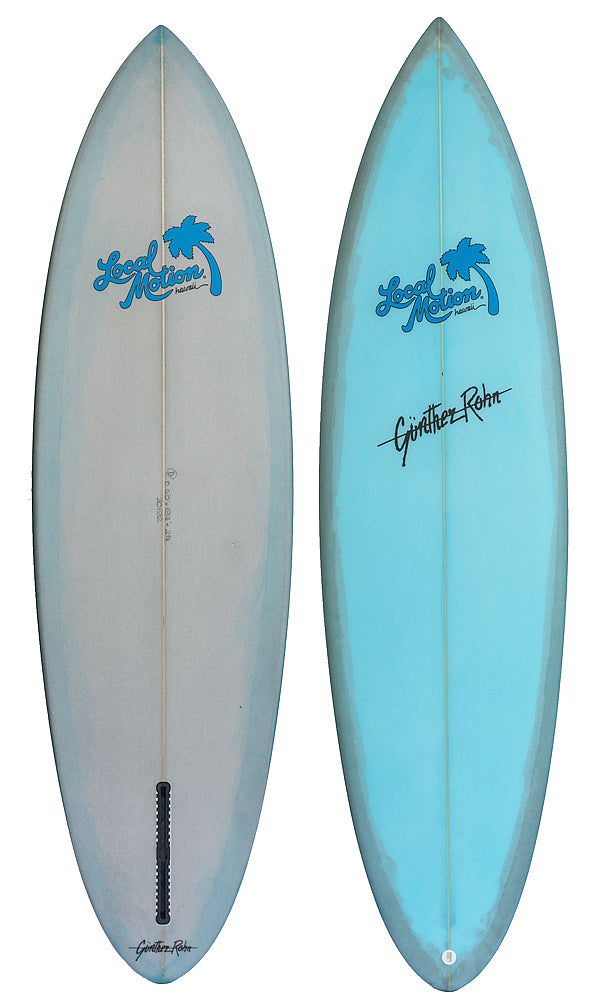This photograph features two surfboards standing upright side by side, both crafted by the brand Local Motion Hawaii. The surfboard on the left is predominantly white with a striking aqua or teal Local Motion logo at the top, accompanied by an aqua or teal cutout of a palm tree. The bottom of this surfboard displays the signature "Gunther Roan." In contrast, the surfboard on the right is an aqua color and mirrors the same Local Motion logo and palm tree design. This board also bears the signature "Gunther Roan," but larger and positioned at an angle in the center, unlike the straight-across signature at the bottom of the white surfboard on the left.